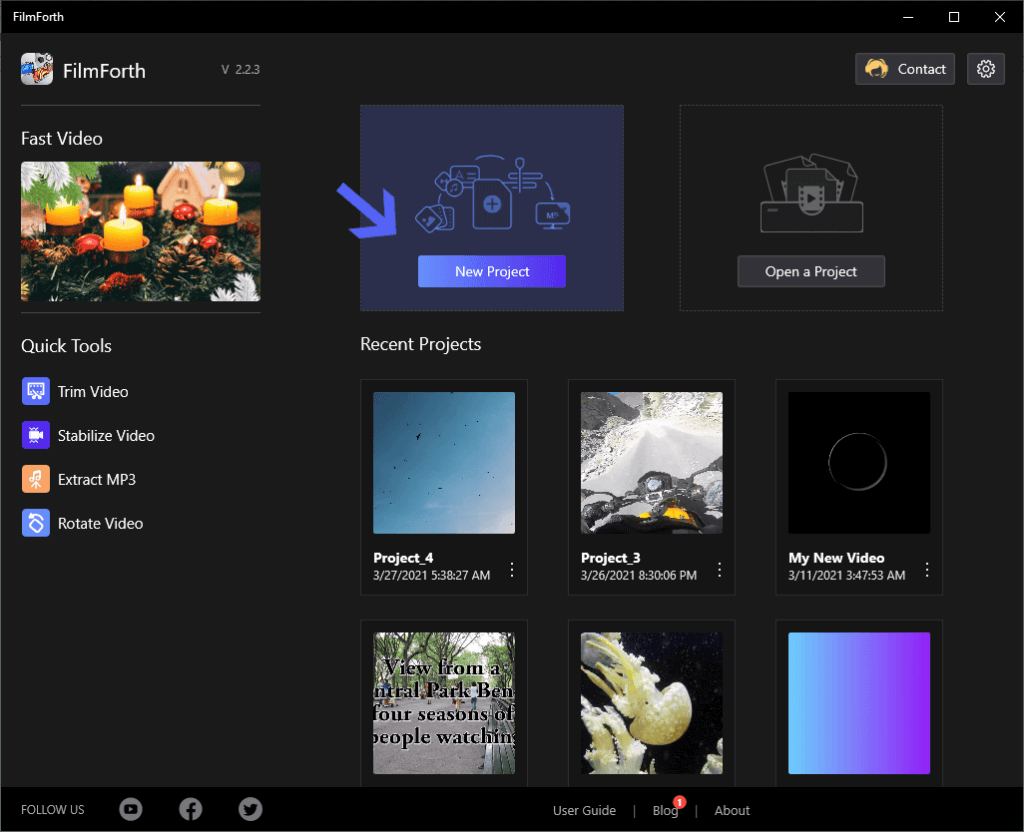This screenshot showcases the main page of a company's software named Filmforth, currently at version 2.2.3. In the top left corner, the Filmforth logo and version number are prominently displayed. The top section provides navigation options, including a contact link and settings configuration.

The primary interface seems to be designed for individual users to manage and create video projects. Key features include options to start a new project, open an existing project, and view recent projects. Below these options, a list of recent projects is visible, including details such as project titles and creation timestamps.

For example, "Project 4" was created on March 27, 2021, at 5:38:27 AM, and features an image of the sky with some clouds. "Project 3," created on March 26, 2021, at 8:30 PM, showcases a person riding a motorcycle in a snowy landscape. Another project titled "My New Video" is also listed, suggesting the platform's robust capabilities for video creation and project management.

On the left side of the interface, against a black background, thumbnail images provide a visual representation of each project. The diversity in these images indicates the versatile nature of the software, catering to various types of multimedia projects.